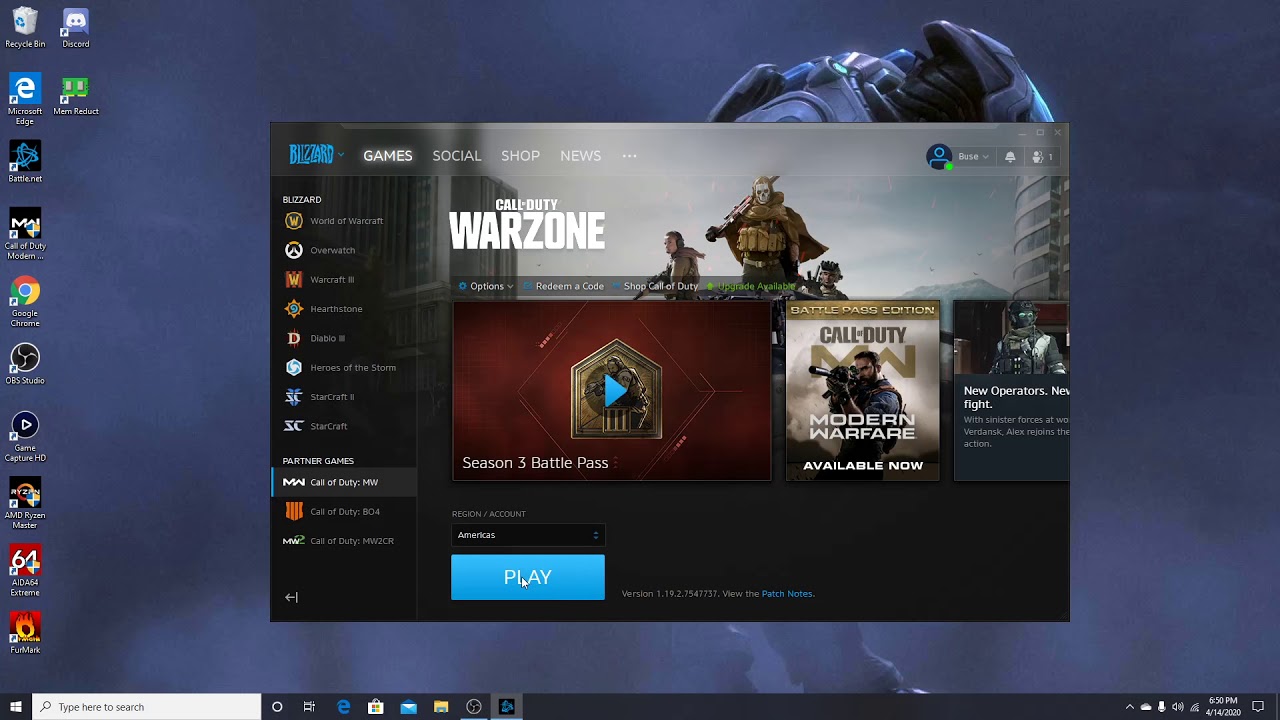The screenshot is a rectangular snapshot of a computer home screen, showcasing a neatly organized arrangement of application icons on the left side of the desktop. At the top-left corner is the Recycle Bin icon, characterized by white text and a gray bin with a blue recycling symbol. Adjacent to it is the square-shaped Discord icon, featuring a white robot face in its center. Following these, a sequence of software icons are aligned vertically: Microsoft Edge, Battle.net, Call of Duty, Google Chrome, OBS Studio, Game Capture, AMD Ryzen Master, AIDA64 Extreme, and Furmark.

Dominating the center of the image is an open application window, identified as the Battle.net interface. The upper-left corner prominently displays the Blizzard logo, rendered in stylized blue letters. The interface showcases a menu on the left, listing various games owned by the user, with adverts prominently featuring Call of Duty: Warzone in the center, distinguished by its white text. The underlying desktop background is dark blue, adorned with imagery of mech armor, which is partially visible behind the open Battle.net window. The overall aesthetic is sleek and organized, providing a clear glimpse into the user's gaming preferences and desktop setup.